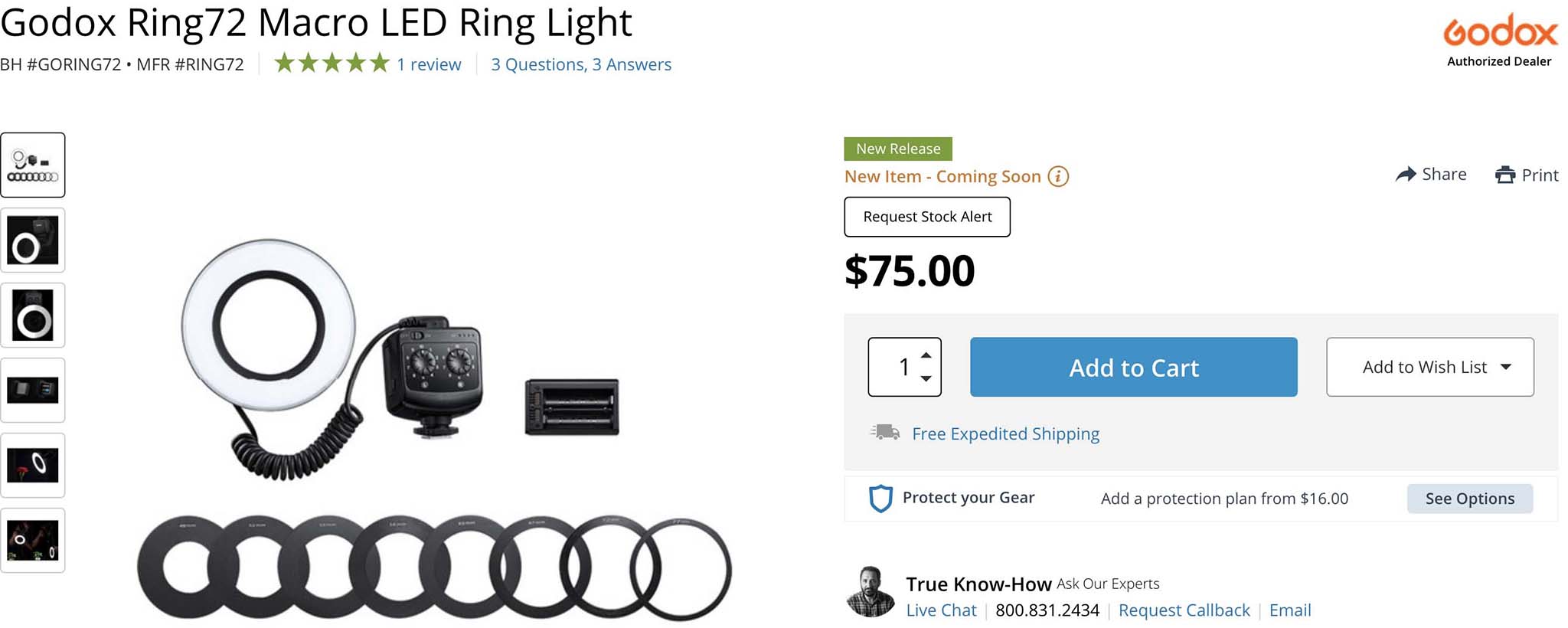This screen capture showcases an online shopping interface for the Godox Ring 72 Macro LED Ring Light, a product frequently used for enhancing lighting in online videos. The interface features a variety of elements typical of an e-commerce product page. 

In the top left corner, the product name, "Godox Ring 72 Macro LED Ring Light," is prominently displayed. The top right corner bears the label "Godox Authorized Dealer," indicating that the website is an official vendor for Godox products. 

The left side of the screen includes a vertical strip of clickable thumbnail images, offering different views and angles of the product. Adjacent to this, slightly left of the center, is a larger, more detailed image of the ring light itself, allowing potential buyers to examine the product closely.

On the right side of the screen, the price of $75 is clearly listed. Below the price are various interactive options, including buttons to "Add to Cart," "Add to Wish List," and other standard shopping actions. Additionally, the interface features an option for live chat support, providing shoppers with immediate assistance if they have any questions about the product.

Overall, the screen capture illustrates a clean and organized online shopping experience, meticulously designed to provide users with all the necessary information and options to make an informed purchasing decision.